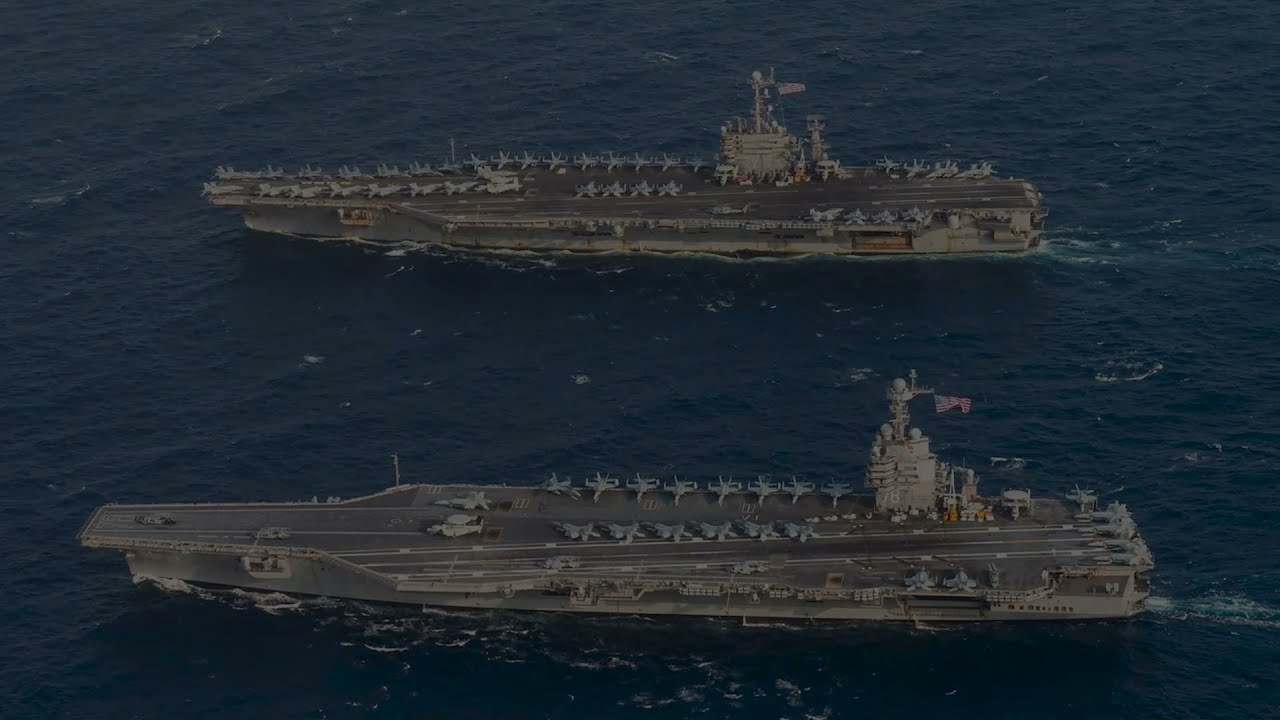This detailed aerial photograph, likely taken from a helicopter or drone, captures two U.S. Navy aircraft carriers sailing side by side on the open sea. These massive, gray vessels, though slightly different in size and model, are virtually parallel as they make their way through the deep blue water. Both carriers are teeming with numerous jets and reconnaissance planes, all lined meticulously along the deck, ready for takeoff. Each ship proudly displays an American flag atop its control tower, positioned approximately three-quarters of the way down the vessel. The image portrays the carriers as they move in unison towards the left side of the frame, against a backdrop of endless ocean, exuding power and precision. The photo appears slightly murky, suggesting potential underexposure, yet it still vividly captures the impressive scene of military might and naval coordination.